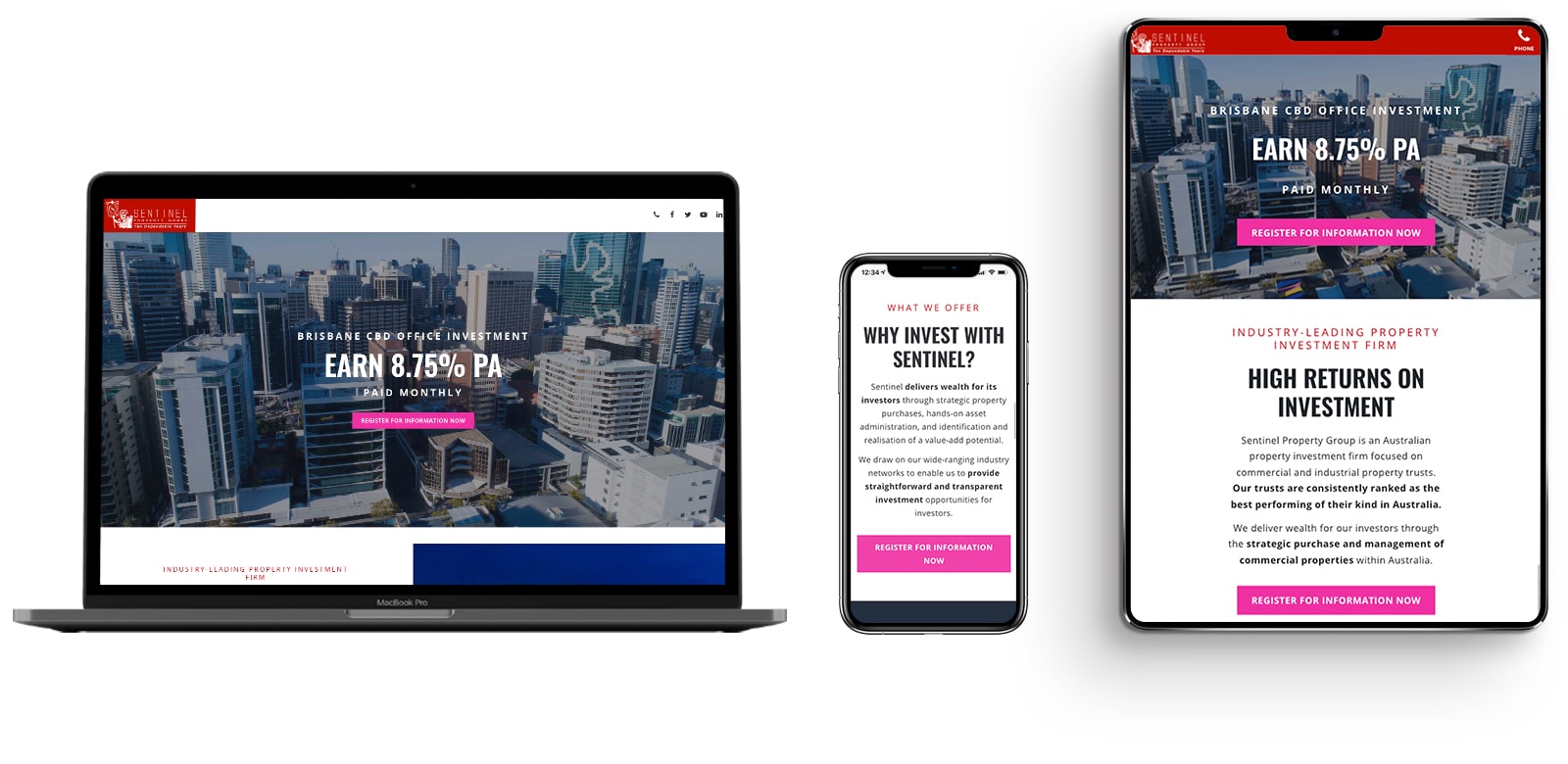In this image, we observe three devices aligned from left to right: a laptop, a smartphone, and a tablet. 

On the left, the laptop screen displays a financial application. The screen reads, "Earn 8.75% PA," with "Earnset 8.7%" prominently featured. The background of the screen showcases an aerial view of a bustling cityscape with numerous skyscrapers. The top left corner of the screen is highlighted in red, while the rest of the top is white. The bottom left section of the screen remains white, transitioning to a blue hue on the bottom right. The laptop's front edge, visible at the base, is gray.

In the center, a smartphone screen catches the eye with the header, "Why Invest with St. Nell," in black text, complemented by pink text at the top. The screen contains two paragraphs of explanatory text in black, beneath which lies a pink rectangle featuring white lettering. The very bottom of the smartphone screen is black.

To the right, a tablet mirrors the same financial information found on the laptop. It displays, "Earn 8.75% PA," with "Earnset 8.7%" over the same city skyscraper backdrop. The top section of the tablet screen is red, and it also contains a pink rectangle in the center. Below this, the text "High Returns on Investment" is clearly written in black, followed by another paragraph in black text. The pink rectangle reappears at the bottom, also containing white text. There is a subtle gray shadow on the left and bottom edges of the tablet, adding depth to its appearance.

This meticulously detailed setup showcases a cohesive financial theme across multiple devices, with a consistent message and design elements.